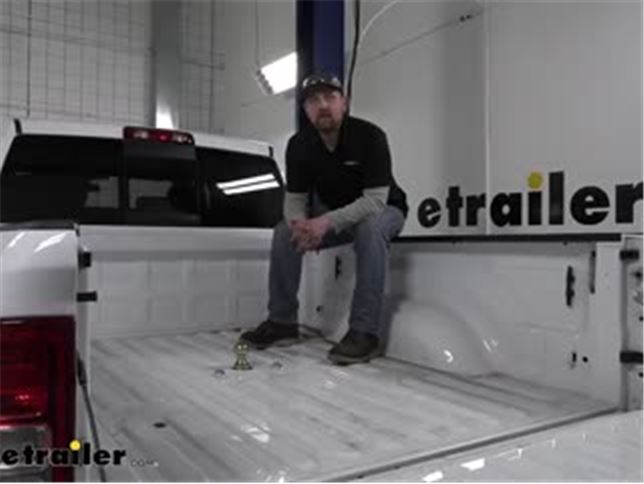In a brightly lit, white-walled garage or warehouse, a bearded man with a mustache sits calmly in the bed of a white pickup truck. The truck features red tail lights, tinted back windows, and a fifth wheel for trailer hauling. The man, wearing gray pants, black shoes, and a dark polo shirt over a long-sleeved gray shirt, dons a black cap with possibly an emblem or sunglasses resting on it. His hands are folded on his lap, and he looks directly at the camera with a neutral expression. Behind him, the wall displays partial lettering that spells out "e-trailer," missing an initial "R." The indoor setting includes distinctive blue beams running down the middle of the space and red bed lights on the cab, contributing to the well-lit ambiance of the photograph.